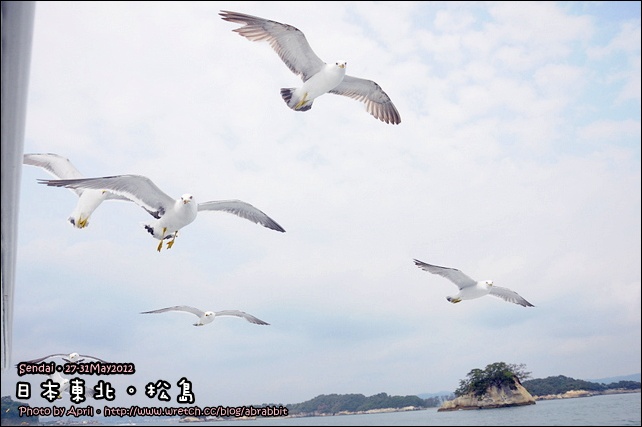The photograph captures five seagulls in flight against a predominantly cloudy sky with occasional patches of blue. The seagulls dominate the scene; two are prominently in focus at the forefront, while the remaining three appear more distant and less detailed. One seagull is notably looking directly at the camera. Beneath the birds, a serene body of water meets the lush, green-capped islands in the distance. The image is framed by a black border, indicative of previous web use, and bears a watermark in the lower left corner. The watermark includes three lines of text: “Sendai + 27-32 MAY2012,” Japanese kanji with wide spacing between characters, and “Photo by April” accompanied by a URL: "http://www.wretch.cc/blog/abrabit."